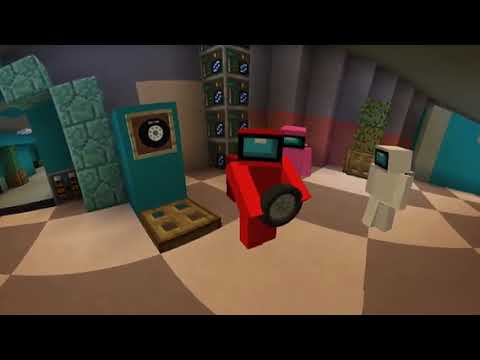This detailed computer-generated image, reminiscent of Minecraft, showcases a room with distinct elements and characters. The scene features a checkered floor with brown and light brown tiles, accompanied by gray walls. Prominent in the foreground is a red, pixelated figure with a TV screen for a face, arms outstretched holding a tire or wheel. This character is flanked by a pink figure and a white figure, both similar in design but not holding any objects.

To the left of the red figure, there's what appears to be a clock on a green slab, followed by a concrete frame or pillar leading to a doorway. Behind the three figures, part of the wall is blue, adorned with what looks like a picture of a tire. Below it is a peculiar brown crate. The background reveals a series of pillars and a tree planted in a container, adding to the room's diverse decorations.

The image's borders are thick and black, framing the Minecraft-like scene. The room includes additional details such as a bluish-gray brick archway on the left. The visual design is highly reminiscent of Among Us characters, each with a visor-like feature in the middle of their TV screen faces, enhancing the blend of familiar gaming aesthetics. The setting appears to be within a base, incorporating various textures and elements like a trapdoor and potted plants, contributing to an intricate and lively environment.